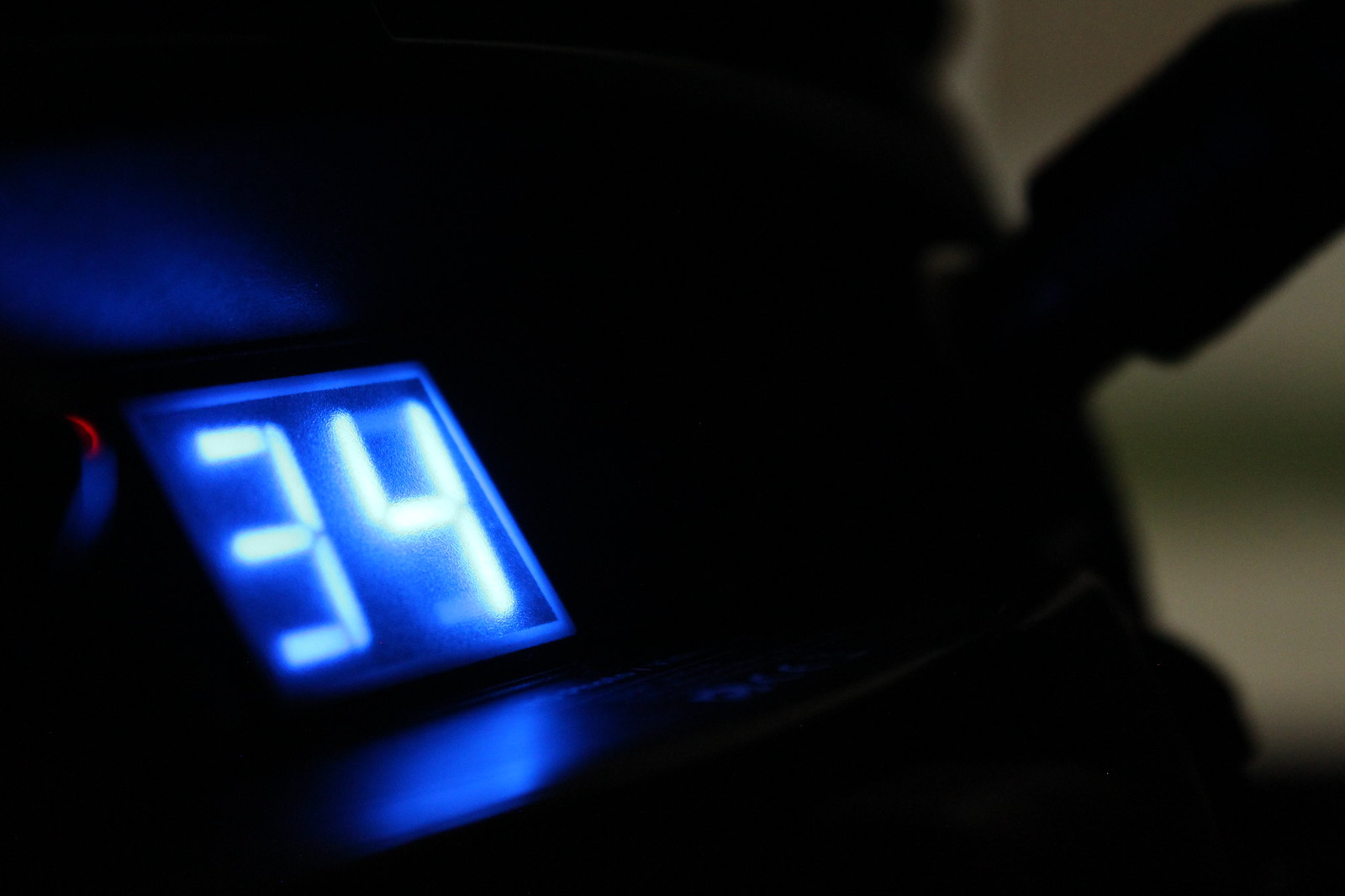This close-up image captures the intricate details of a black digital device, likely a thermostat. The digital display is centered in the foreground, showcasing the number "34" prominently within a square display box. There's a noticeable glare in the upper section of the display, hinting at a blue light source. Additional illumination in red and blurry blue hues is visible on the left side, adding contrast to the color scheme. A lever is situated in the upper right-hand corner, indicating a manual control component. The device's surface beneath the digital display reflects a blue tint, enhancing the visual intricacy of the image. The background is intentionally kept blurry, focusing the viewer’s attention on the device's detailed features.